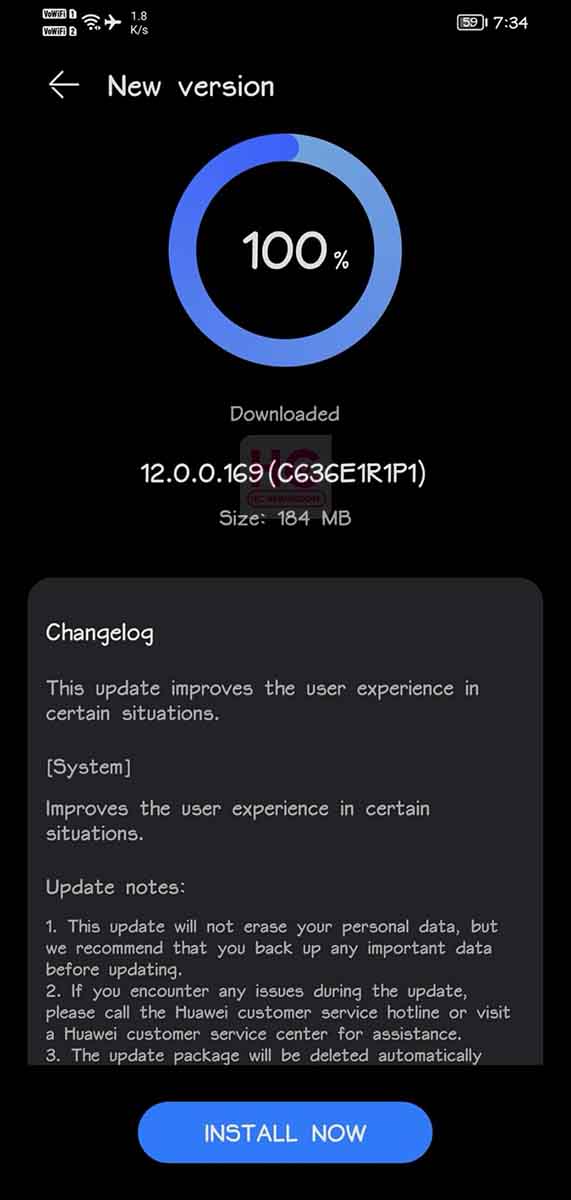The image displays a smartphone screen against a solid black background. In the top left corner, various small icons indicate the phone is in flight mode and has an active WiFi connection. On the right, it shows the battery at 59% and the time at 7:34 in white text. Below this, on the left side, there is a left-pointing arrow accompanied by the text "New version." 

Beneath this, a circular icon depicts a blue line that progressively darkens as it completes the circle, with "100%" displayed in the center. Below this circle, it states "Downloaded: Version 12.0.0.169, Size: 184 MB."

A grey panel follows, with "Changelog" as its heading in white text. This section details the update's enhancements, including improved user experience in certain situations, and provides system information along with various update notes enumerated as 0.1, 0.2, 0.3, etc. At the very bottom, a blue button with white text reads "Install now."